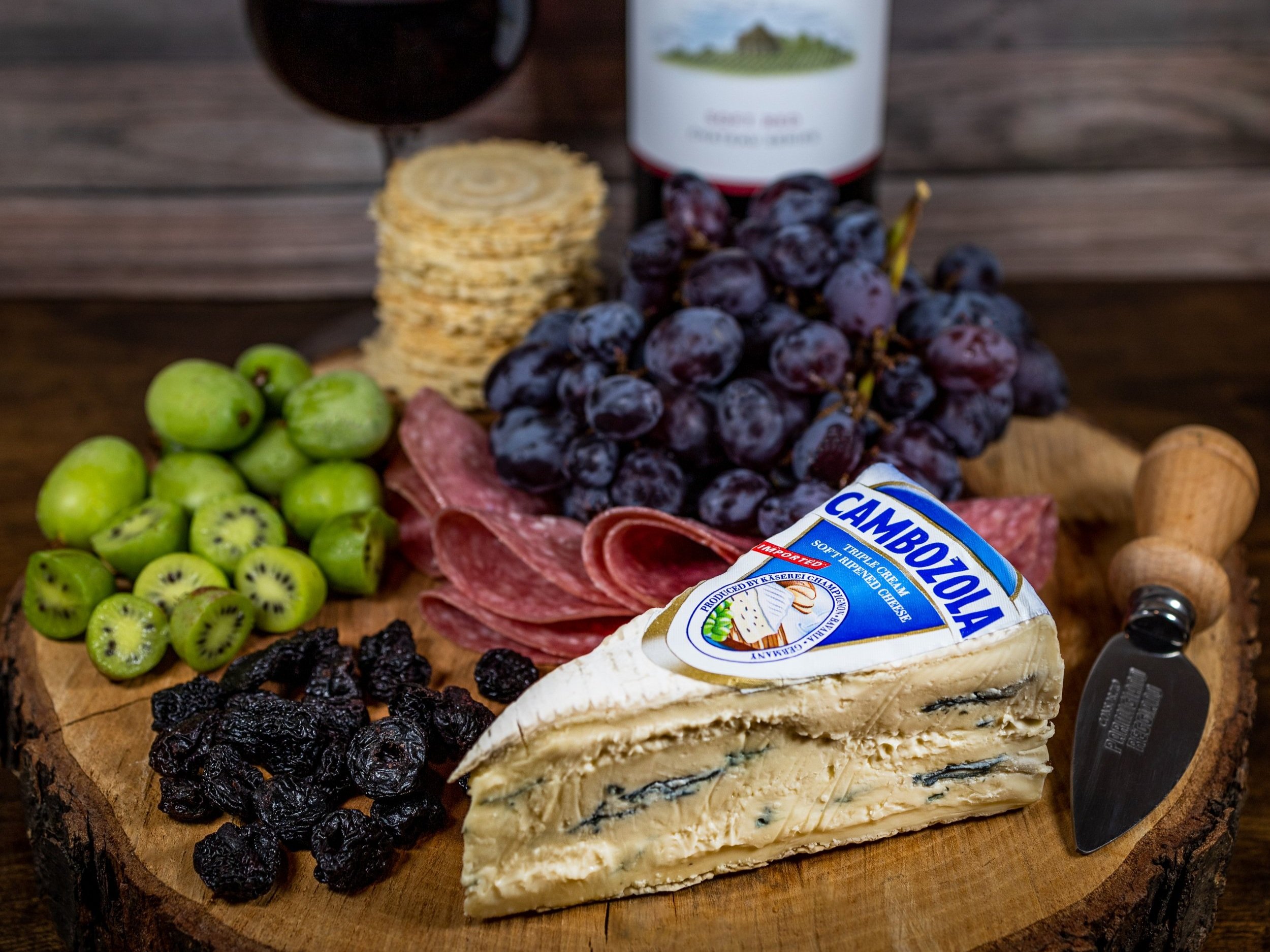The photograph captures a detailed charcuterie board artfully arranged on what appears to be a slice of a tree stump, serving as a rustic platter. Dominating the foreground is a large wedge of Cambozola triple cream soft ripened cheese, bearing a clear label. Directly to its left, there is a grouping of fresh raspberries. Adjacent to the raspberries are several green fruits resembling kiwi, some sliced and some whole. A stack of swirly crackers is situated behind the kiwis, contributing to the board’s diverse texture. To the right of the crackers, a bunch of dark purple-red grapes is elegantly draped over a stack of folded salami or similar cured meats. Adding to the ensemble is a cheese knife placed on the right side. In the blurred background, a bottle of red wine and a glass can be discerned, enhancing the gourmet ambiance. The scene is set against a backdrop of wooden slats, emphasizing the rustic theme of the presentation.